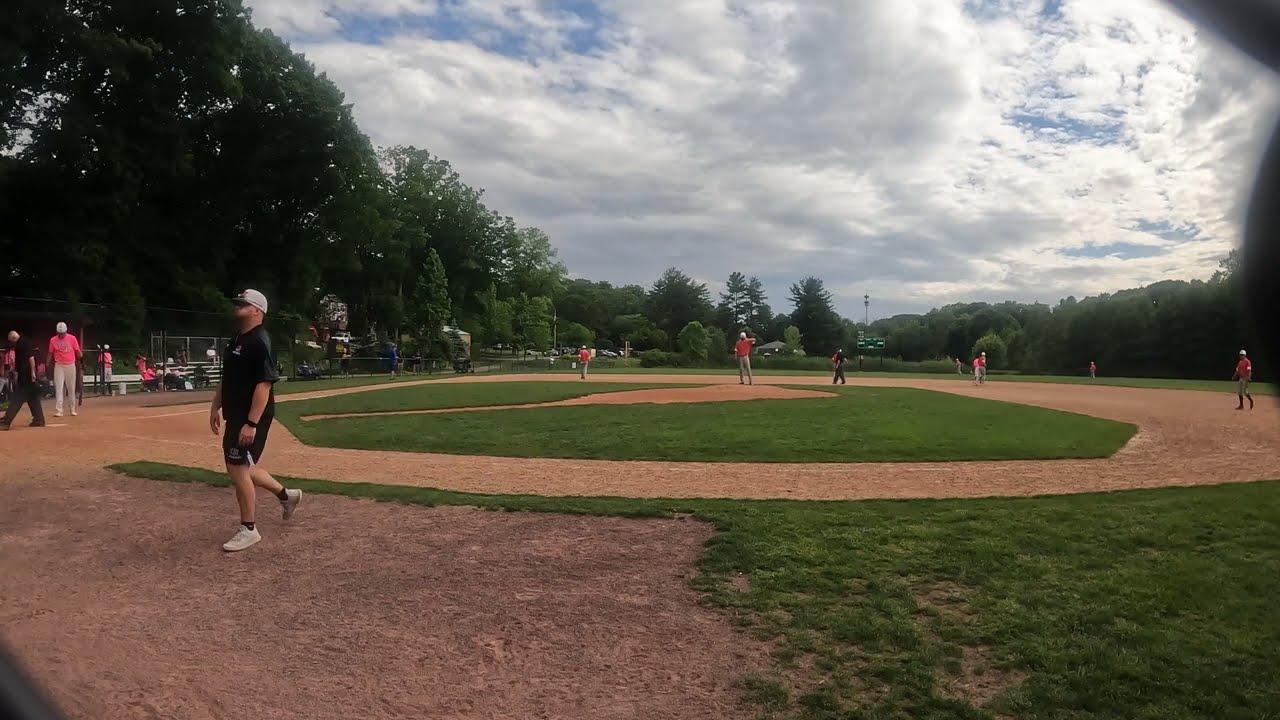The image depicts a local park baseball diamond bustling with activity during a cloudy daytime. In the foreground, a middle-aged man wearing a black shirt, black shorts, white sneakers, and a white cap is walking away from the field, possibly a coach. The field, surrounded by pine trees and other greenery, showcases players in distinct team uniforms: one team in bright orange tops with white caps and white pants, another team in blue jerseys with gray pants. Two umpires are visible, one positioned behind home plate, ready for the incoming batter, and another possibly stationed between second and third base. On the left side of the frame, there is a relatively empty bench for the orange team, with most players out in the field. Key players are visible, including an approaching batter and a pitcher on the mound. The well-maintained field, with its clay surface and clearly delineated baselines, extends into a background where houses and parked cars are partially visible. The sky, filled with cumulus clouds, suggests this photo was taken late in the afternoon.